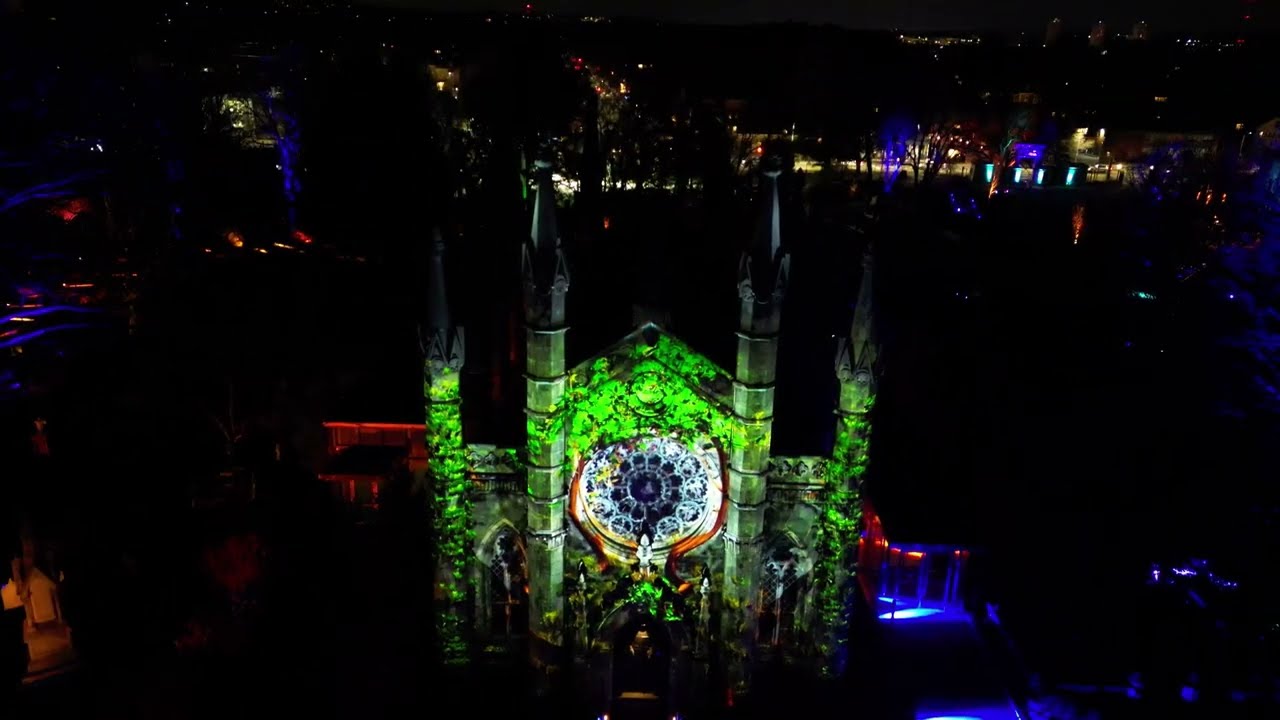This photograph captures the facade of an ornate cathedral at night, brilliantly illuminated by vibrant green, blue, and white lights. The cathedral's front, framed perfectly in the center of the image, features four tall round pillars; the two central pillars rise higher than the outer pair. Dominating the middle of the structure is a grand, circular gothic window, bathing in a mix of white and blue light that almost resembles an 'evil eye.' The green lights cast onto the stone facade create an organic, scientific blob-like pattern, adding a surreal touch to the scene. The surrounding cityscape fades into the darkness but is dotted with scattered variously colored lights, including bluish glows near the cathedral and reddish lights further away. White streetlights line a distant road, complementing the occasional yellowish light spots presumably from buildings or vehicles. Despite the ambient lights, the background remains largely indiscernible due to the overwhelming darkness, amplifying the cathedral’s luminous prominence.